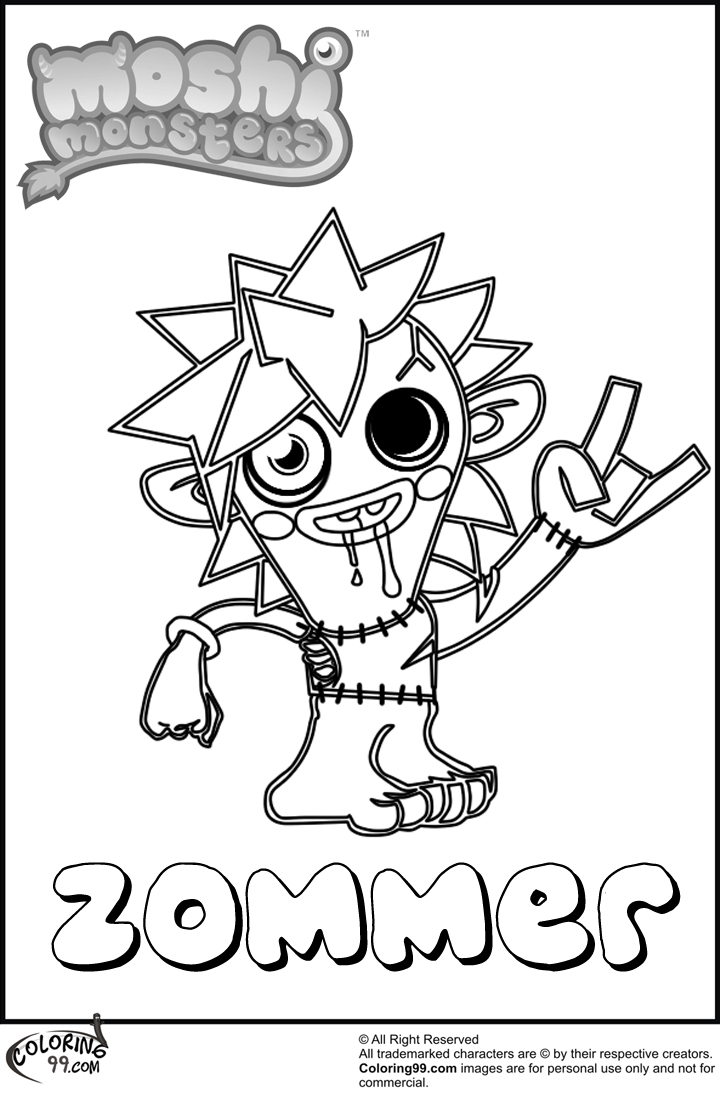The image is a black-and-white cartoon drawing featuring a whimsical monster character associated with Moshi Monsters. The monster, identified as "Zommer," is depicted with spiky, unruly hair and asymmetrical, exaggerated eyes—one eye is a completely black circle, while the other is more typical with an iris. The creature's mouth is a gaping semicircle, from which drool visibly drips, and it sports just two prominent teeth. Zommer's appearance is further embellished with stitching around its neck, wrists, and torso, suggesting a patchwork or Frankenstein-like assembly. Adding to its playful demeanor, Zommer is shown flashing a peace sign with one hand while appearing barefoot and clad in a simple t-shirt. The image features the Moshi Monsters logo in the top left corner and the name "Zommer" in bubbly lettering at the bottom, with a mention of the website Coloring99.com in the lower left corner.